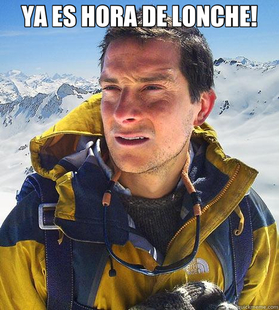In the image, a very muscular man with a short-cropped beard and shaved head, resembling a professional wrestler, is seen kneeling on a bed. He is wearing nothing but a jockstrap, revealing his bare buttocks, and has a black tattoo on his right shoulder. The man is grasping a black cylindrical pillow with white stripes, positioned between his legs. Surrounding him are black pleather pillows also adorned with white stripes. The bed is dressed with a comforter featuring a camouflage pattern in shades of gray, black, white, and red, alongside a black under sheet. The headboard is a dark brown wood with posts on either side, framing the bed against a dark gray wall. Electrical outlets are visible on both sides of the bed. Dominating the center of the image are the bold white letters "H-A-I" in impact font with a black border, giving the impression that the photograph could be part of a meme.